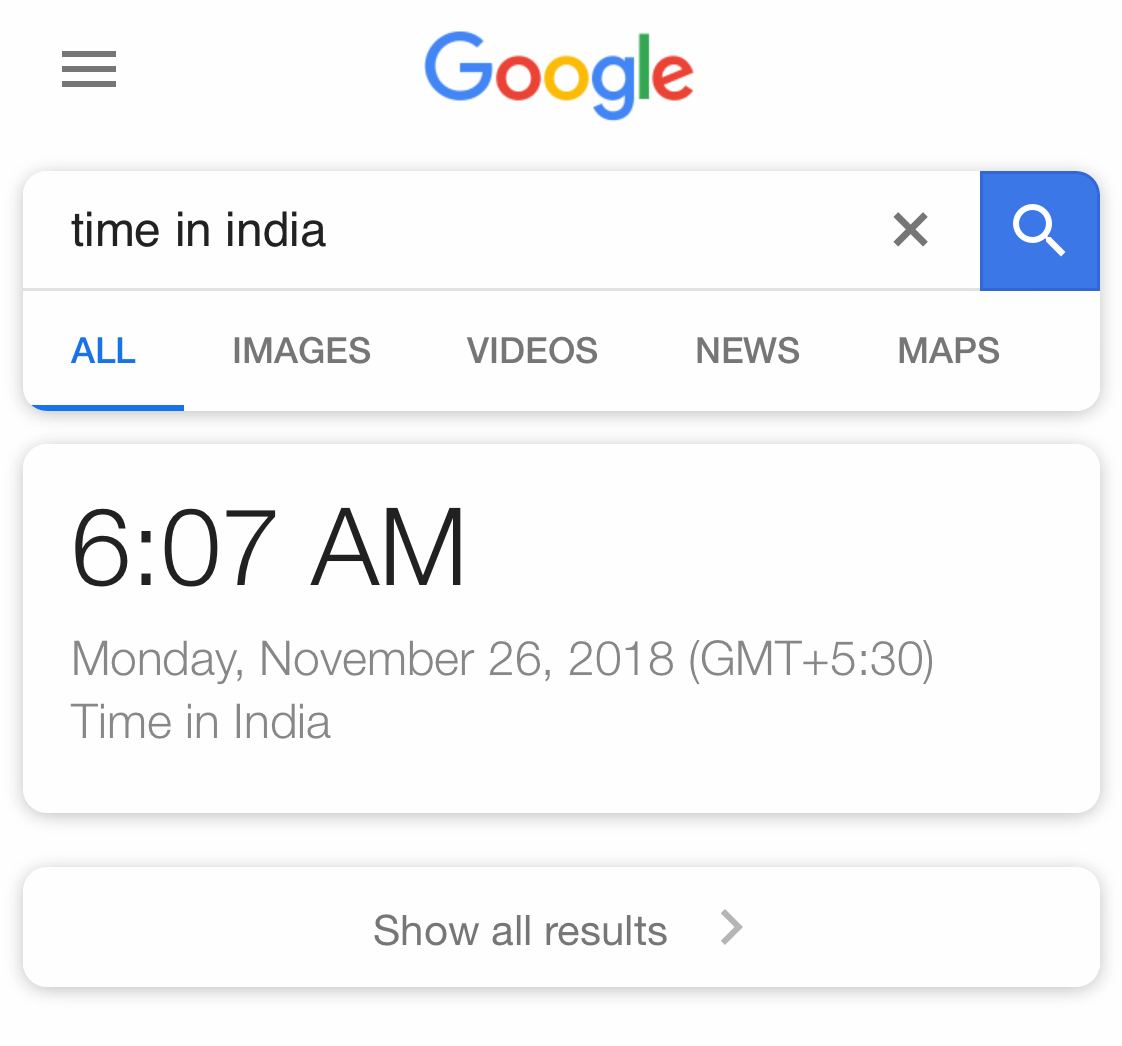This detailed image depicts a cropped screenshot of a Google search results page. The background is predominantly white. 

In the top left corner, there is a dark gray hamburger menu icon. Central to the top section of the image, the multicolored Google logo is prominently displayed with a capital blue "G," a lowercase red "o," a yellow "o," a blue "g," a green "l," and a red "e." 

Beneath this logo is a white, rectangular search bar with rounded corners. Inside the search bar, positioned towards the top left, "time in India" is typed in black text. The search bar is bisected by a thin light gray line. On the far right end of the search bar, there is a dark gray "X" button. To the right of this button, a blue square with a rounded top right corner contains a white magnifying glass icon.

Below the search bar, a row of navigation options is displayed. These options include "All," "Images," "Videos," "News," and "Maps," with "All" highlighted in blue and underlined, while the rest are in dark gray. This navigation bar casts a faint medium gray shadow.

Directly beneath this navigation row, a larger pane contains key information. In the top left, large black text displays "6:07 AM," followed by light gray text beneath it indicating "Monday, November 26, 2018," and in parentheses, "GMT+5:30." Further down, in justified left alignment, additional black text reiterates "time in India."

Below this pane, a narrower section contains medium gray text in the center that reads "Show all results." To the right of this text and following a small area of empty space, there is a dark gray arrow pointing to the right toward more empty space.